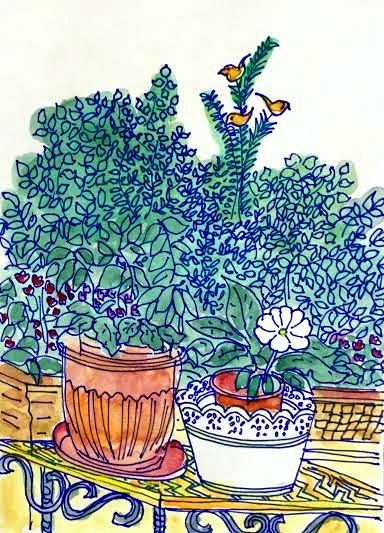This image showcases a captivating mixed-media painting that masterfully combines ink and watercolor. The artist demonstrates exceptional skill in blending and layering the paints, creating a rich and textured composition. The artwork features an intricate scene where the initial outlines of vibrant green blobs suggest lush foliage. These outlines have been meticulously detailed with a dark blue pen, adding depth and precision to the piece. The scene comes to life with meticulously rendered leaves, pots adorning a tabletop, and a couple of delicate birds perched on the branches. The harmonious use of water and ink reveals the artist's profound understanding and command over their materials, resulting in a visually striking and impressive painting.